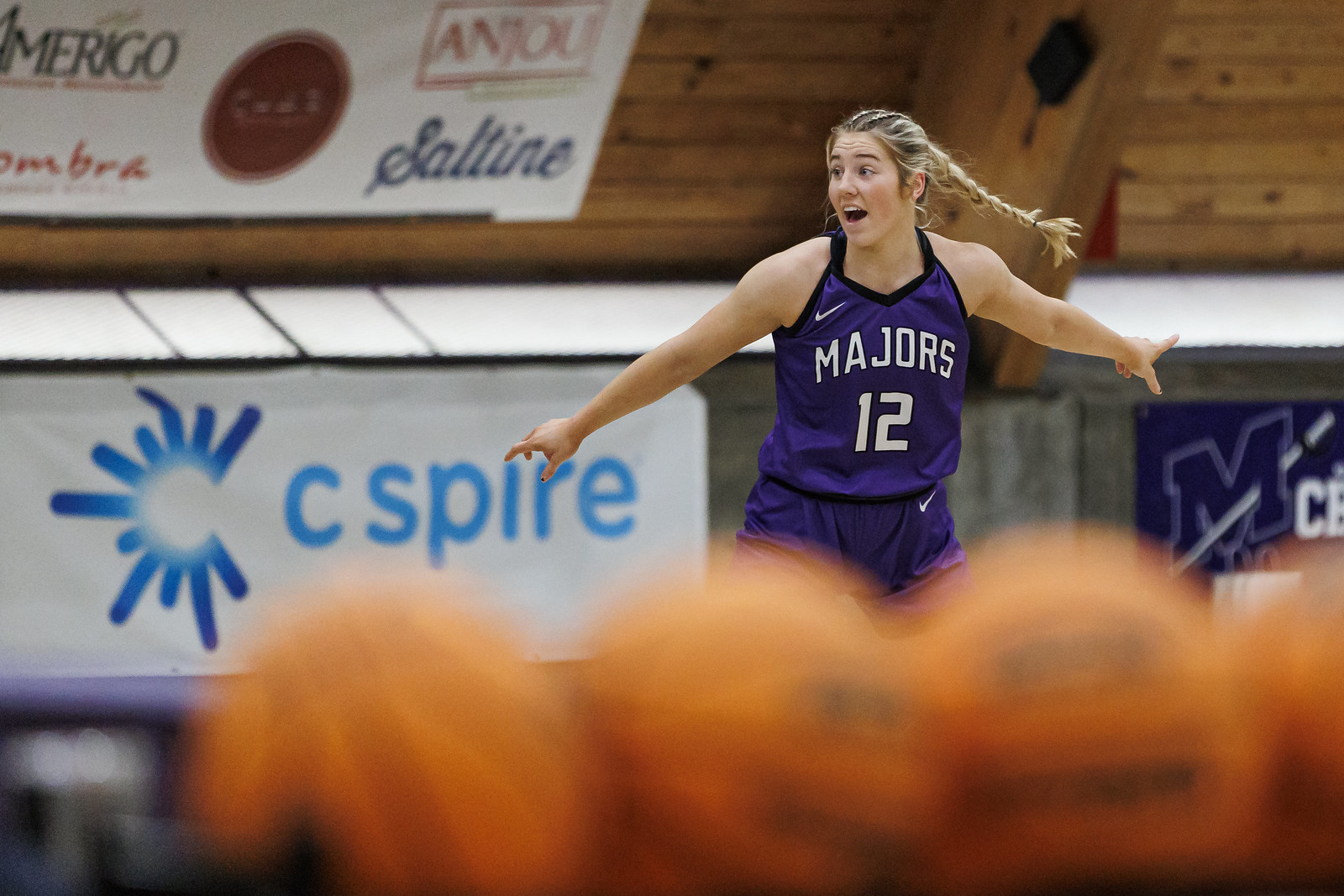This is a dynamic indoor action photograph of a Caucasian female basketball player, likely in her late teens or early 20s. She is positioned slightly right of center, with her arms extended outward in a defensive stance and her mouth open in what appears to be happy surprise, suggesting she just made a significant play. Her blonde hair is pulled back into a long braided ponytail that flies behind her head, further emphasizing the action of the moment.

She is wearing a dark purple basketball uniform, with a tank top and matching shorts. Across the chest of the tank top is "MAJORS" written in white curved lettering, accompanied by the numerals "12" below it. A white Nike logo is placed just above the "M" in "MAJORS" on her jersey and another on her right hip of her shorts. 

The setting is an indoor basketball court with a planked wooden ceiling and an arched beam. Various sponsorship banners, including ones that say "C Spire," "Anju," "Saltine," "Amerigo," and "Sombra," adorn the background. In the foreground, partially covering the girl's legs, is a row of blurry, orange basketballs, giving depth to the image while keeping the focus on the player. The entire image is a horizontal rectangle, capturing the essence of an intense moment within the game.